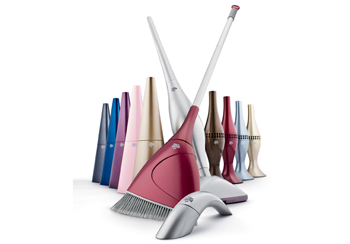The image appears to be a professionally edited photo, likely used for advertising various cleaning products. Central to the image is a unique broom with violet bristles, standing out amidst a diverse array of cleaning tools. Surrounding the broom is an assortment of what appears to be handheld vacuums or other compact cleaning instruments, meticulously arranged in V-shaped rows extending from the foreground to the background. These tools come in an array of colors, including bronze, blue, red, black, gold, maroon, turquoise, pink, and silver. The photo's backdrop is a stark white, enhancing the vivid hues of the products, and there is no text present in the image. The overall setup and sleek design of these items suggest a space-age aesthetic, simultaneously functional and visually appealing, perfectly suited for a contemporary advertisement of modern cleaning supplies.